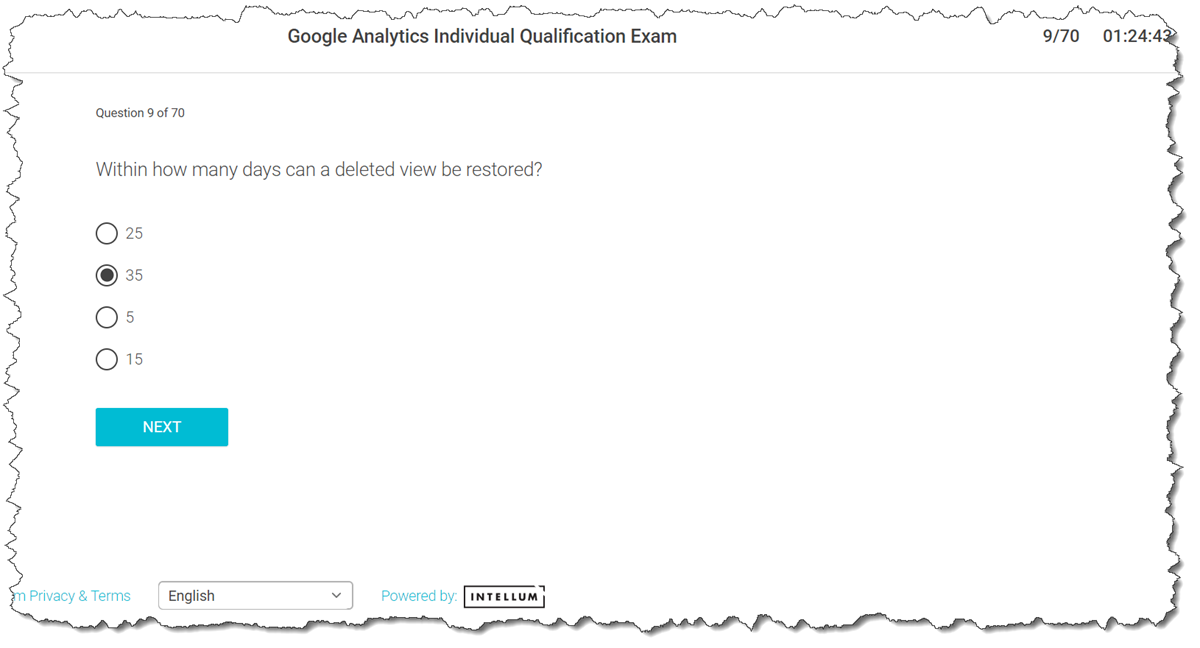This image is a detailed screenshot from the Google Analytics Individual Qualification Exam interface. The page exhibits question 9 out of a total of 70, with the timestamp indicating the user has spent 1 hour, 24 minutes, and 42-43 seconds on the exam so far. The visual presents a unique "ripped paper" effect around its borders, adding an artistic flair to the screenshot.

The question displayed on the screen is: "Within how many days can a deleted view be restored?" The multiple-choice options provided are 25, 35, 5, and 15 days, with the choice of 35 days currently selected by the respondent. However, it is noted that 15 days is also highlighted, possibly indicating a previous selection.

Below the question and answers, a teal-colored square button labeled "Next" is visible, prompting the user to proceed to the subsequent question. Near the bottom of the interface, text reading "Privacy and Terms" along with a dropdown menu to select the English language is present, enhancing the page's accessibility. Additionally, towards the lower center, there is a notation that reads "Powered by Intellum," acknowledging the platform supporting the exam.

This screenshot provides a comprehensive visual record of the exam interface and user interaction, capturing various elements and design details.